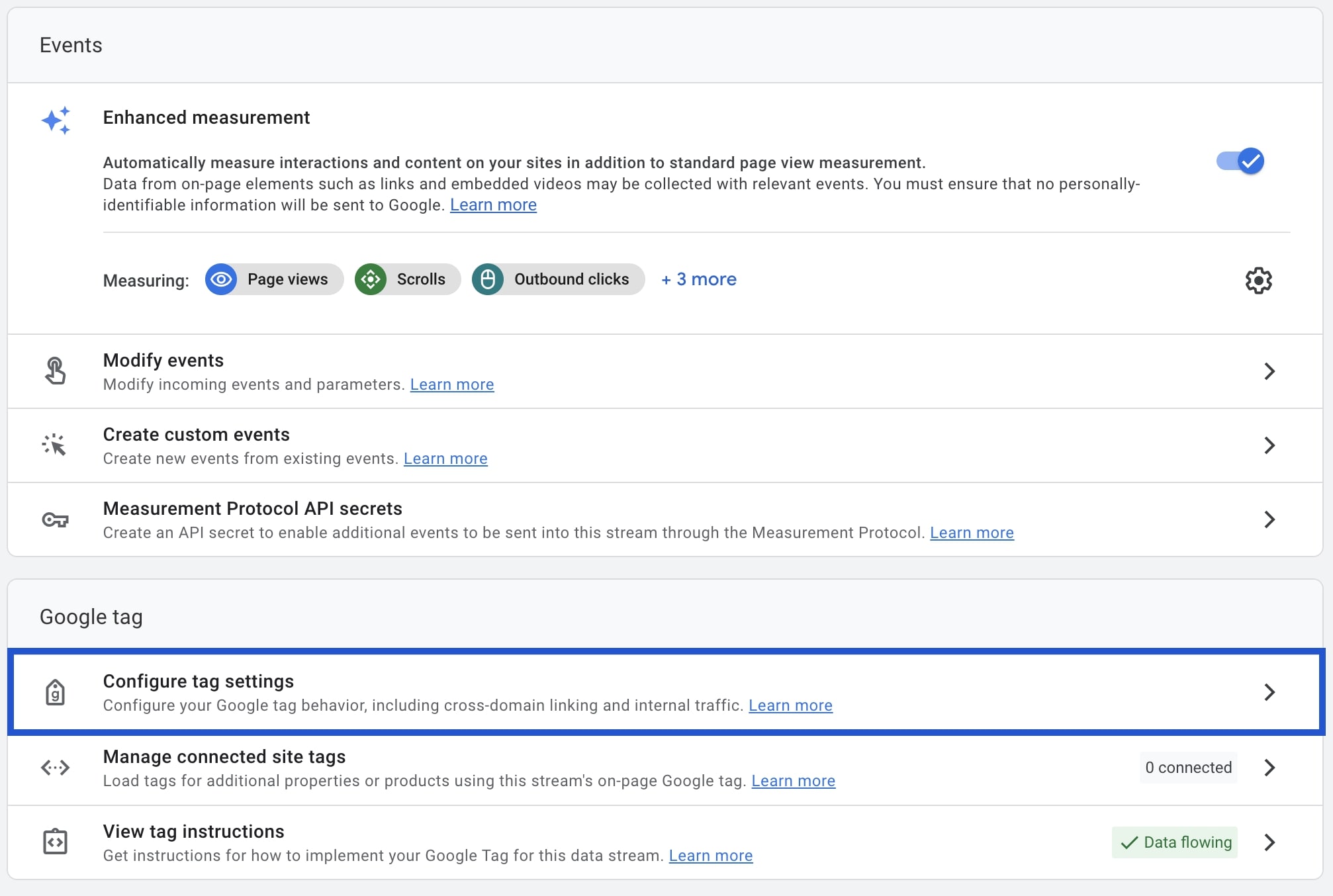The image depicts a detailed interface of a web management page for Google, used as a hosting platform for websites. At the top of the page, there is a section labeled "Events," accompanied by a three-star logo indicating a high rating for the website. Directly below, there's a description about the "Enhanced Measurement" feature, which automatically tracks interactions and content on the site beyond standard page view metrics. It mentions that data from page elements, such as links and embedded videos, are collected as relevant events. A reminder is included to ensure no personally identifiable information (PII) is sent to Google for privacy compliance.

Beneath this section, the word "Measuring" is prominently displayed, followed by several rounded rectangles with colored circle icons along their left edges. These icons represent different metrics: Page Views, Scrolls, and Outbound Clicks, with an indication that there are three more metrics available. To the far right of this row, a gear icon represents the Settings option.

A horizontal rule divides this from the next section which includes "Modify Events" with an arrow suggesting a pop-out menu. This section allows users to "Create Custom Events" and manage "Measurement Protocol API Secrets," enabling additional events to be routed into the data stream through the measurement profile.

Further down, the hierarchical structure lists "Google Tag." A blue rectangle highlights an item within this list, specifically "Configure Tag Settings," which allows configuration of Google Tag behaviors such as cross-domain linking and internal traffic management. Below this, there are options to "Manage Connected Site Tags" and "View Tag Instructions," providing comprehensive tools for managing and understanding the application of Google Tags on the website.